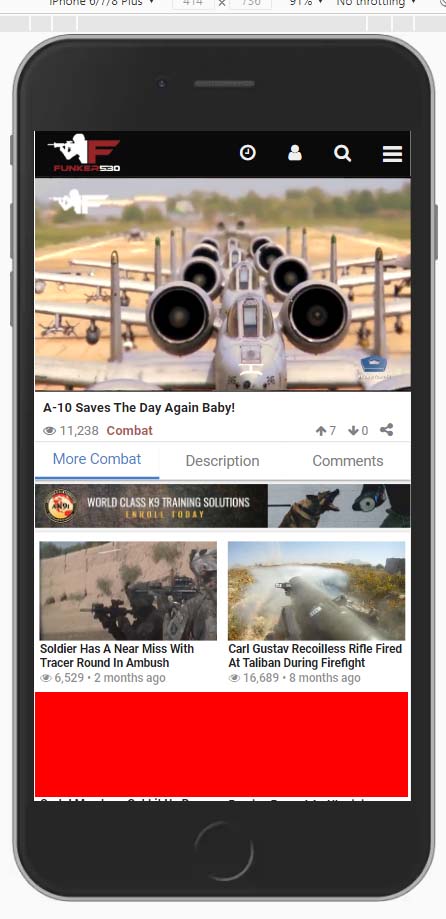A screenshot of a cell phone, fully visible with its casing. The phone's casing is a sleek, steel gray color surrounding the screen. At the top of the screen, there is a familiar black bar typical of many cell phones. Below this, a black banner spans the width of the screen featuring distinct icons and text.

On the left side of this banner, there's a white icon resembling a soldier aiming a rifle. To the right of this icon, the left side of a large red "F" is prominently displayed. Beneath the "F" is some red text that is illegible, followed by "530" in white. Towards the right side of the banner, there are three icons in white: a clock, a person, and a search icon. Further to the right, there are three horizontal white lines stacked one atop the other.

Below this banner, an image depicts a lineup of fighter jets positioned in a row on an airstrip, with trees visible in the background. The title beneath the image reads, "A-10 saves the day again, baby," accompanied by a gray figure "11,238" and the word "combat" in red. The post has received seven upvotes, zero downvotes, and includes a share button.

Below this section, there are three labels: "more combat" in blue (currently selected), "description" in gray, and "comments" in gray. Underneath these labels, there are a series of images with captions. One image is labeled "world-class K-9 training solutions," showing a dog being trained by a person in heavy padding.

Further down, two equally sized images are displayed. The left image is captioned "soldier has a near miss with tracer round in ambush," and the right image is titled "Carl Gustav recoilless rifle fired at Taliban during firefight."

At the very bottom of the screen, there is a large red bar, and beneath this, the black part of the phone casing is visible.